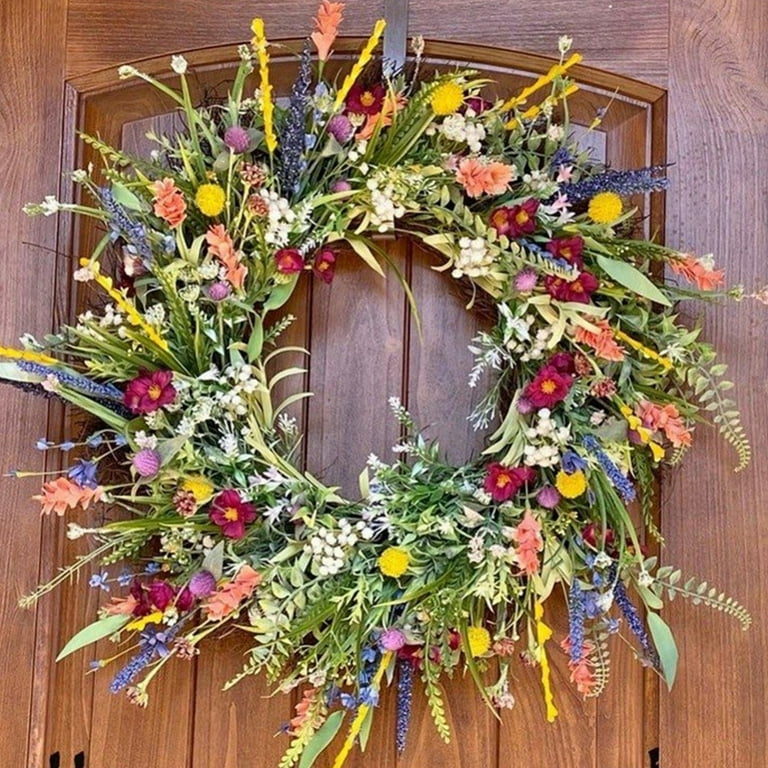The image features a stunning wreath of artificial flowers mounted on a richly polished, medium brown wooden door. The wood displays a distinct grain pattern and panels designed for expansion, giving the door an elegant, almost internal feel. The wreath is a vibrant, polychromatic arrangement with shades of yellow, red, peach, pink, salmon, lilac, lavender, violet, blue, and white flowers interspersed with green leaves and stems. The flowers are arranged in a balanced, circular, and somewhat wispy fashion, creating a dynamic 3D effect. The hardware on the door is black iron, contributing to its refined appearance. A metal strap, likely used to hang the wreath, extends out of the frame. The overall presentation is very lively, well-maintained, and exquisitely detailed, highlighting both the beauty of the wreath and the sophistication of the door.